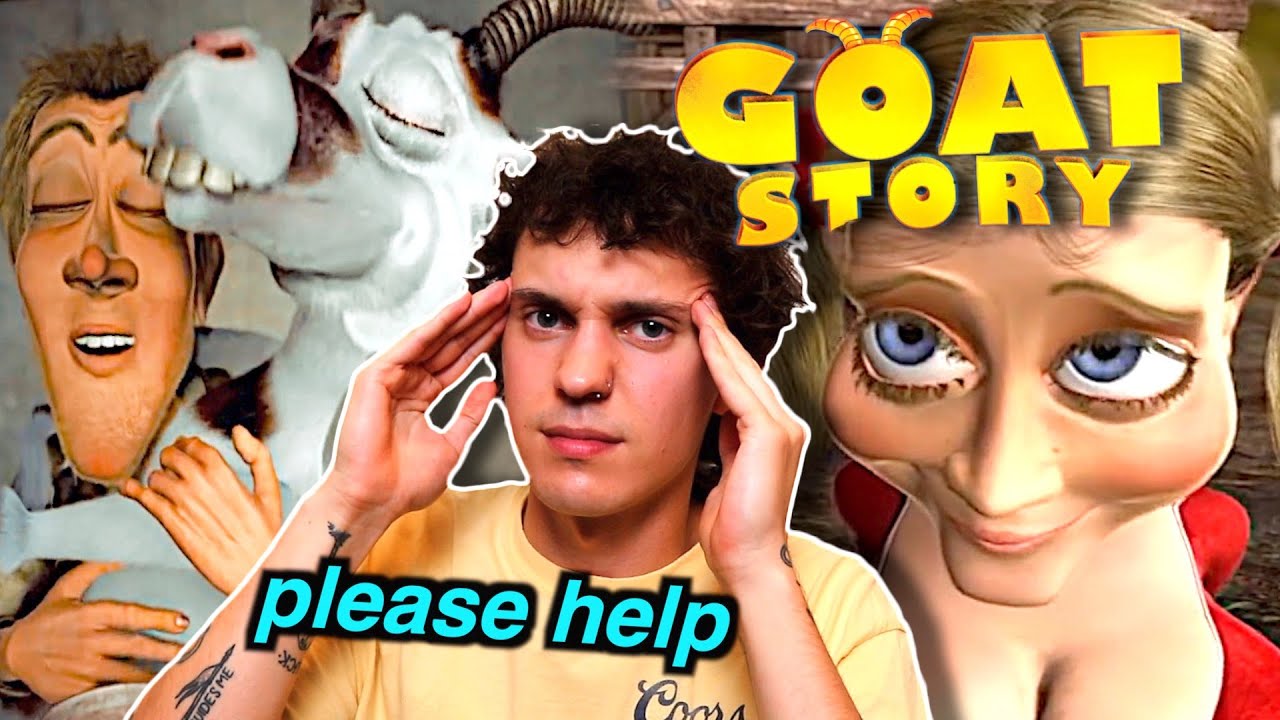This landscape mode image appears to be a montage, possibly a part of an intro video or a screenshot. The top right corner prominently features the title "Goat Story" in bold, yellow text with two goat horns sprouting from the "O". The composition is divided into three main sections. 

On the left, there's a cartoon drawing of a light-skinned man embracing a white goat with brown spots and large horns. Both the man's and the goat's eyes are closed, and the man displays a wide smile, displaying his teeth. His face is exaggerated in a caricature style. 

In the center, a real-life photograph of a light-skinned man with dark, fluffy hair is superimposed. He looks concerned, holding both temples with his fingers, as if experiencing a headache. He wears a yellow T-shirt that says "Kors" and has visible tattoos on his right arm. Overlaid on the photograph, in teal letters, are the words "please help".

On the right, there's another cartoon illustration featuring a blonde, light-skinned woman with pronounced cheekbones, large blue eyes, and wearing a red dress with a deep neckline. Her expression and details are highly stylized, fitting with the caricature theme.

The unique combination of real-life photography and cartoon illustrations, paired with the expressive and bold text elements, builds a striking visual narrative central to "Goat Story".